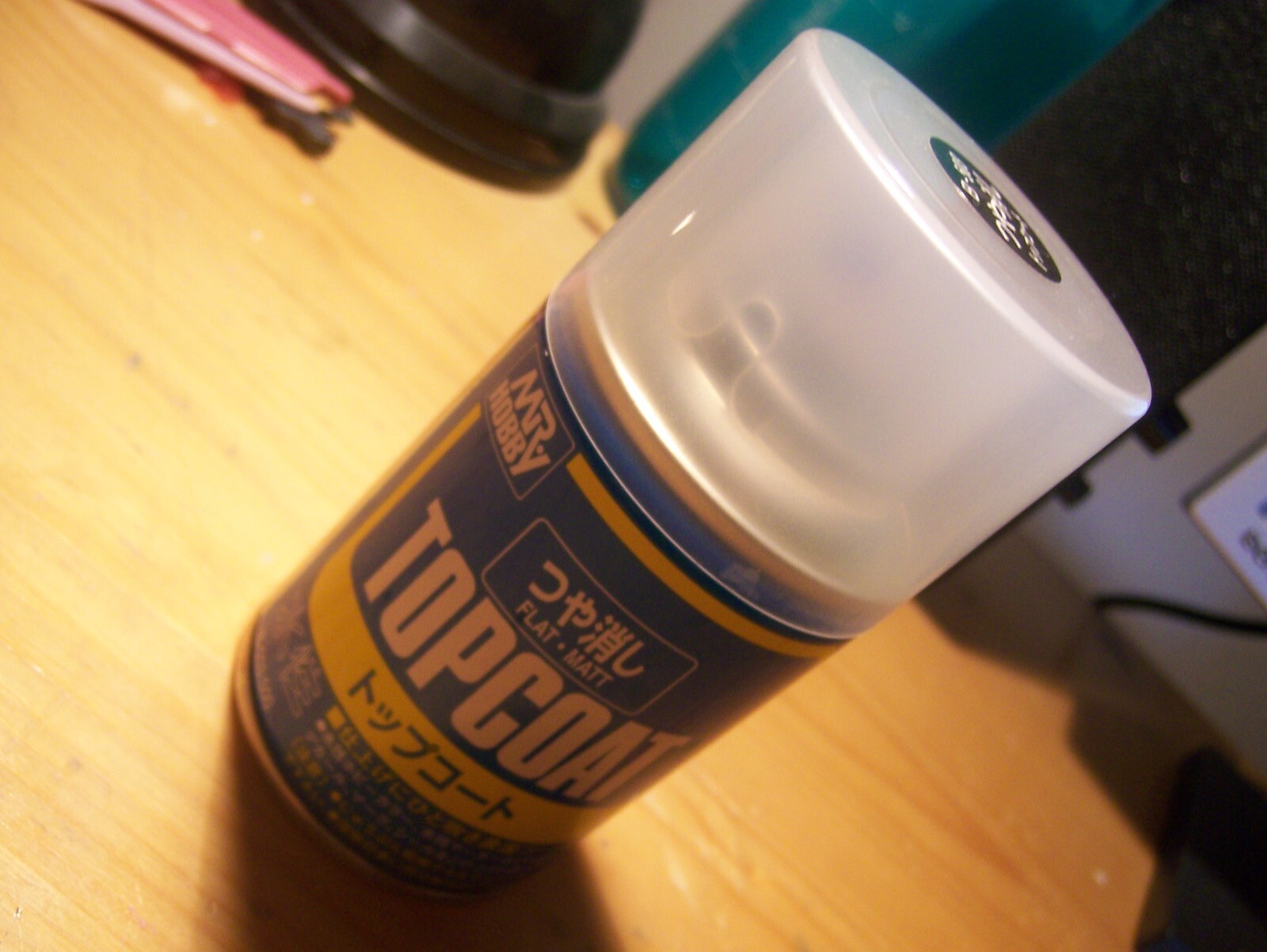The photograph depicts a small spray can of paint placed on a light-colored wooden surface. The can features a semi-transparent clear plastic cap that reveals an inner cylinder beneath it. The main body of the can is blue with white text prominently displaying "Mr. Hobby" and "Topcoat" in large letters. Additionally, there are Asian characters—likely Japanese or Chinese—on the can, some of which are written in white on the blue base, as well as in black on a yellow banner. The image is captured at an angle, giving an odd, tilted perspective of the can leaning over. In the background, a book stands upright, accompanied by glasses and possibly a bowl, further enhancing the setting.